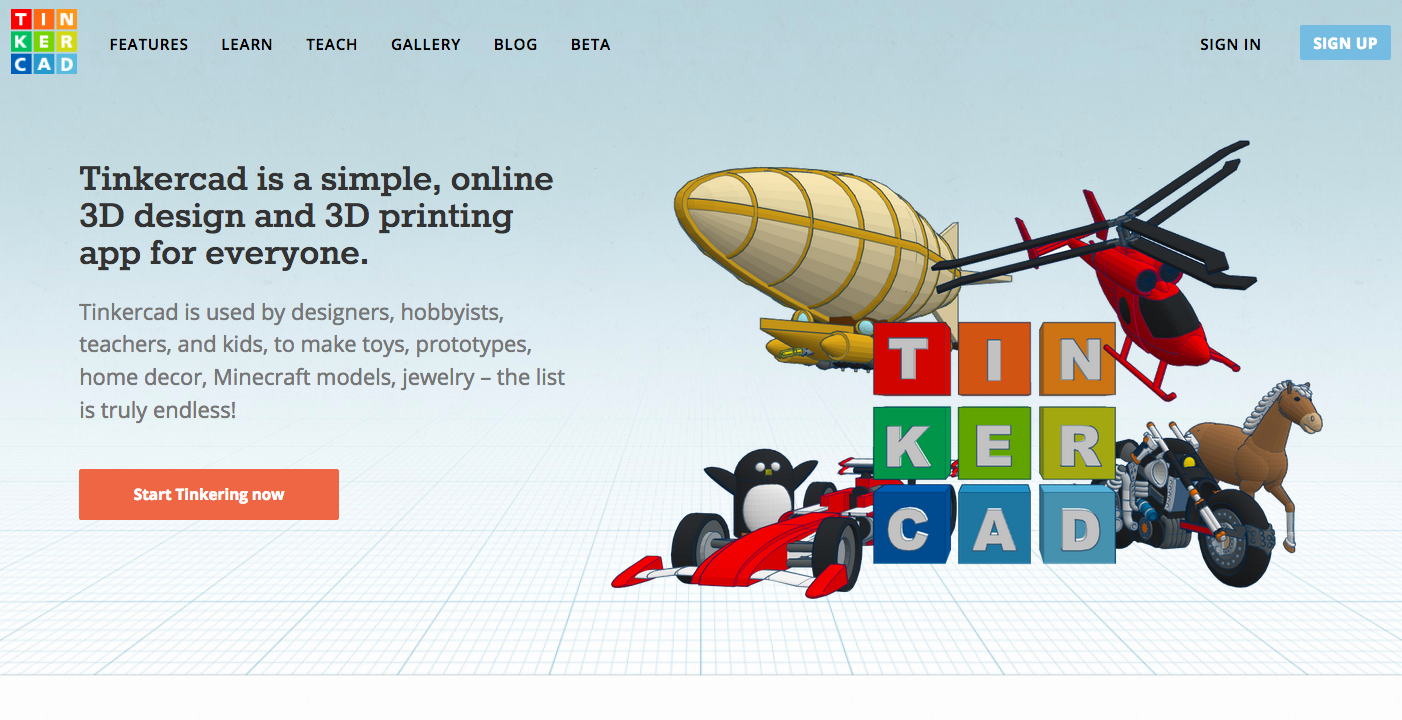The image is a screenshot from the Tinkercad website, displayed in landscape mode as it would appear on a laptop or computer monitor. The background color is a pale sky blue, providing a calming and neutral canvas for the vibrant elements on the page. 

In the top left corner is Tinkercad's colorful logo, which is composed of three rows and three columns of squares, each containing one white letter. The top row spells out "TIN" in red, red-orange, and orange squares. The middle row spells "CUR" in green, lighter green, and yellow squares. The bottom row spells "CAD" in blue, lighter blue, and even lighter blue squares. Together, they form the word "TINKERCAD."

To the right of the logo, a black menu bar lists the following items in bold capital letters: Features, Learn, Teach, Gallery, Blog, and Beta. On the far right of this menu bar, the "Sign In" option is available for existing users, while new users are encouraged to "Sign Up" through a large blue button with white text.

The right-half of the screen prominently showcases an enlarged version of the Tinkercad logo against a background resembling graph paper. Surrounding this logo are various whimsical design elements: a wooden blimp, a red helicopter, a brown horse galloping toward the right, and a matching motorcycle. On the left side of the logo, a penguin with raised wings appears alongside a dragster reminiscent of Formula One racing cars.

The left side of the page contains text introducing Tinkercad, boldly declaring in black letters: "Tinkercad is a simple online 3D design and 3D printing app for everyone." Below this headline, a smaller, non-bolded blurb explains, "Tinkercad is used by designers, hobbyists, teachers, and kids to make toys, prototypes, home decor, Minecraft models, jewelry. The list is truly endless!" 

Finally, a large red rectangular button at the bottom prompts users to "Start Tinkering Now!" inviting them to begin exploring the creative possibilities offered by Tinkercad.